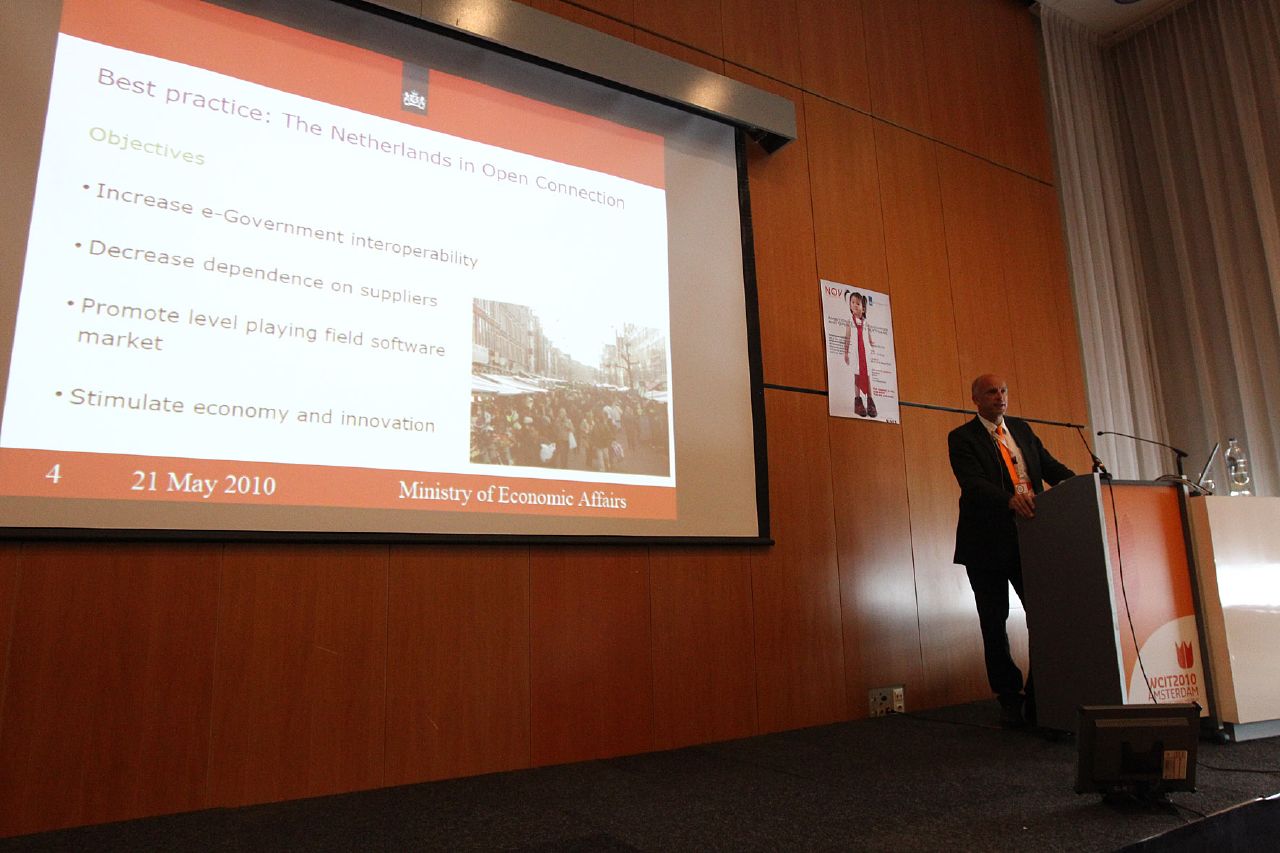In this full-color indoor photograph taken on May 21, 2010, in the Netherlands, a man stands at a wooden lectern giving a lecture. The photograph is horizontally triangular and features a gentleman in a dark suit with a white shirt and a yellow-orange tie. He has very short hair or is bald. Behind him, a large wooden-paneled wall and white curtains are visible to the right. The floor is covered in dark blue or gray carpeting.

The man is positioned towards the bottom right corner of the image. He stands behind a podium adorned with two microphones and a large water bottle. On the back wall, a large projector screen displays a PowerPoint slide. The slide reads, "Best Practice, the Netherlands in Open Connection" and lists objectives such as "increase e-government interoperability, decrease dependence on suppliers, promote level playing field software market, and stimulate economy and innovation." The bottom of the slide includes the date, "May 21, 2010," and mentions the "Ministry of Economic Affairs." Behind the man is also a white poster featuring a little girl, although the details of the poster are unclear. There is a monitor on the floor next to the lectern, presumably for the speaker to reference during his presentation.